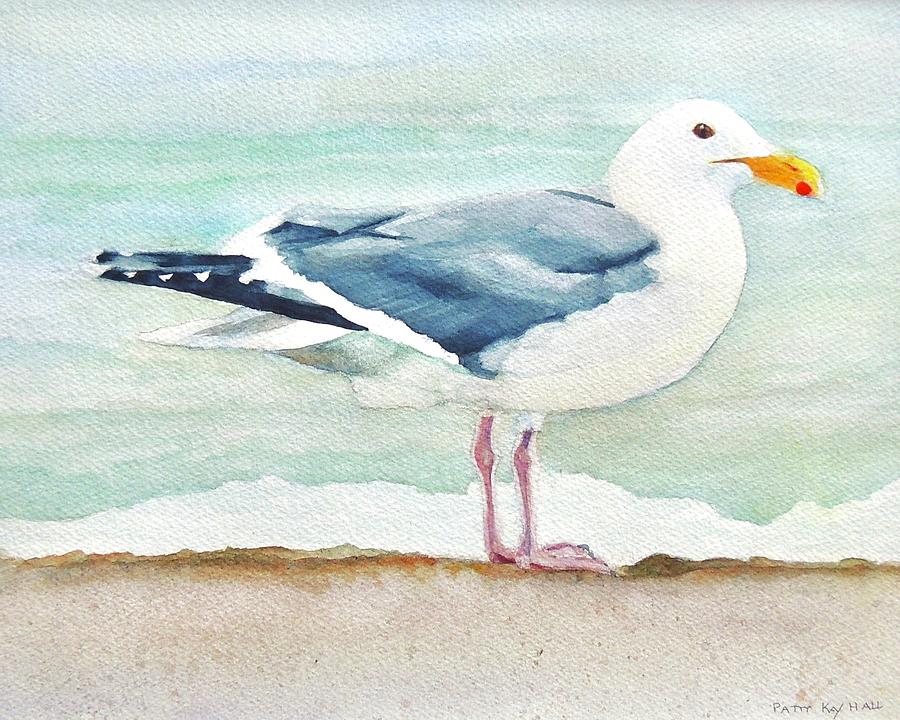The painting showcases a seagull standing upright on a light tan sandy beach. The seagull, positioned centrally and facing right, is predominantly white with a bright yellow-orange beak adorned with a red dot on its tip. Its legs are a pinkish-brown hue, and the wings are gray, matching the gray and white tail feathers. In the background, the blue sky or water creates a tranquil setting, with small waves of green-blue water lapping near the bird's feet. The beach scene, framed with details of the ocean or sky, is subtly signed by the artist in the bottom right corner as "Perry K. Hall."